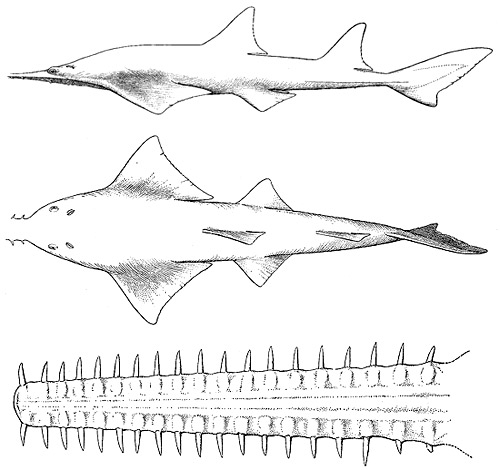This detailed sketch showcases three distinct perspectives of a shark, each meticulously rendered in gray and white. At the top of the image, a side view of a shark reveals a pointed snout and two dorsal fins, with a pronounced rear fin on the right. Positioned directly below, a top-down view of what appears to be the same shark provides a clearer look at its dorsal and side fins, enhancing the viewer's understanding of its anatomical structure. The bottom section of the illustration features what looks like the tail or possibly the specialized head of a hammerhead shark, exhibiting sharp, serrated edges reminiscent of weaponized teeth. This area displays a textured body part, further amplifying the detail and realism of the depiction. The background remains a stark white, ensuring that the viewer's focus remains on the intricate shark illustrations.